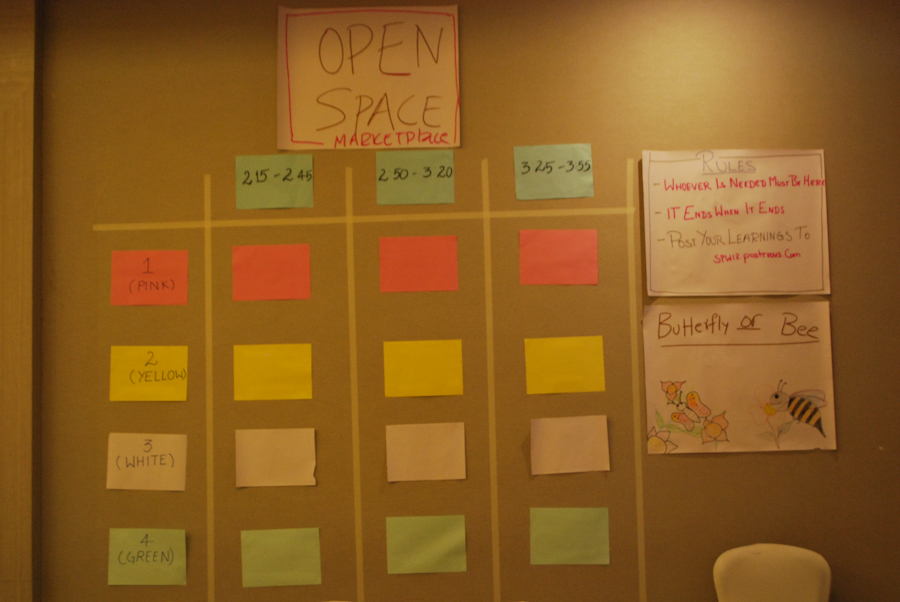This indoor color photograph is of a light brown cork bulletin board prominently displaying various organized items. At the very top, a piece of paper with the header "Open Space Marketplace" stands out. Below it, there are neatly arranged Post-it notes in multiple columns, each column topped with labels in differing colors: green, pink, yellow, white, and green once more. The notes form thorough rows, creating a colorful and structured appearance.

To the right of these notes, two larger pieces of paper are pinned to the board. The first document, titled "Rules," provides guidelines, stating, "Whoever is needed must be here. It ends when it ends. Post your learnings to..." followed by an email address. Directly below the rules, another sheet titled "Butterfly or Bee" features illustrated images of a butterfly and a bee, adding a visual element to the instructional content.

This detailed setup suggests a collaborative working environment, possibly for brainstorming or project management, where openness and participation are emphasized.